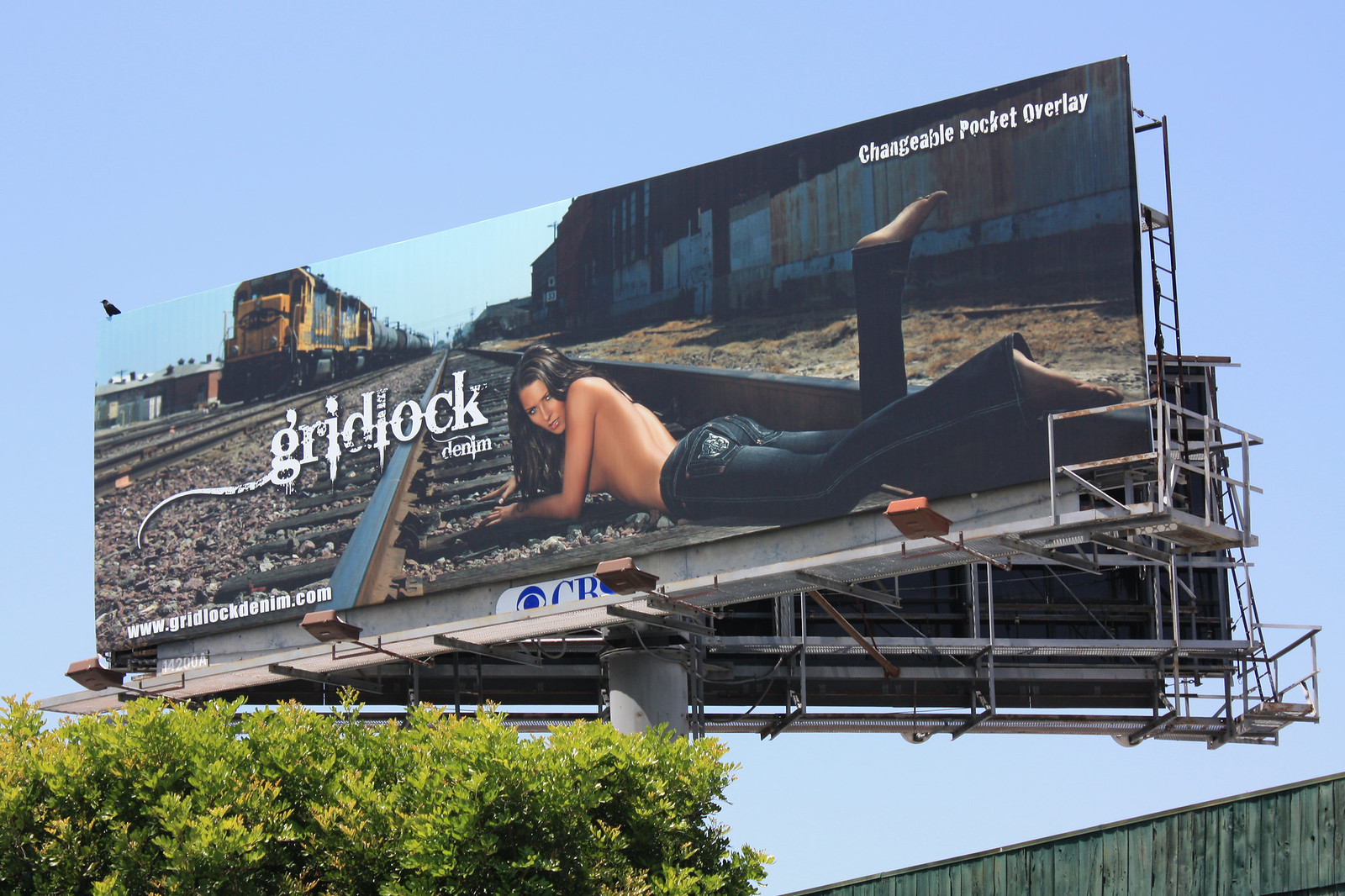This detailed photograph showcases a large billboard advertising Gridlock Denim. The billboard prominently features a topless woman with long black hair, lying on her stomach on a set of train tracks. She is wearing a pair of Gridlock Denim jeans, which stand out with a noticeable stitching pattern on the back pocket. The advertising text includes "Gridlock Denim" next to the woman's head, "Changeable Pocket Overlay" at the top right corner, and the URL "www.gridlockdenim.com" at the bottom left. 

To the left of the billboard's train tracks, a blue and yellow, possibly Santa Fe, locomotive is either parked or directed towards the viewer on a parallel set of tracks. The billboard itself is part of a larger structure, with a second billboard angled away in the opposite direction. The environment around the tracks includes an old industrial building made of corrugated metal and a large, tall fence running alongside the tracks. In the upper left corner of the billboard, a bird is depicted facing off to the side. The overall scene is set against a clear blue sky with no clouds, and the lighting suggests midday sun, enhancing visibility. The ground beneath the billboard is obscured, but lush green shrubbery can be seen just below the sign's lower rail, where the logo "CBS" is printed. The ad is eye-catching yet controversial due to the dangerous setting depicted for the model.